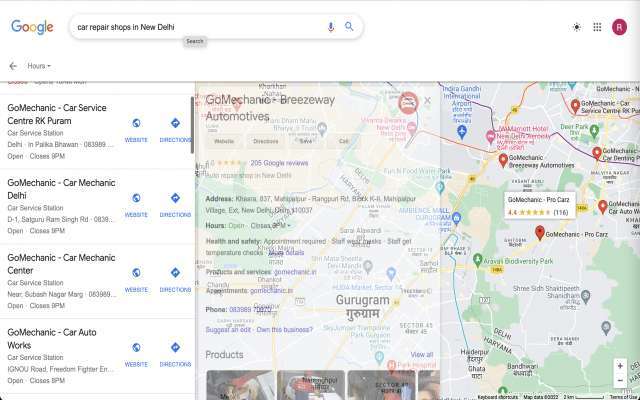The image depicts the search results page of Google. At the top of the page, right beside the Google logo in the search bar, the query "Car Repair Shops in New Delhi" is visible. The first search result is labeled "Go Mechanic Car Service Center R.K. Puram," and subsequent results include "Go Mechanic Car Mechanic Delhi," "Go Mechanic Car Mechanic Center," and "Go Mechanic Car Auto Works." Each entry is identified as a "Car Service Station." Though slightly blurry, the image reveals that beneath each shop's name, their respective addresses and operating hours are listed, indicating they all close at an unspecified time in the PM. To the right of the search results is a map displaying the locations of the listed car repair shops, marked for easy identification.